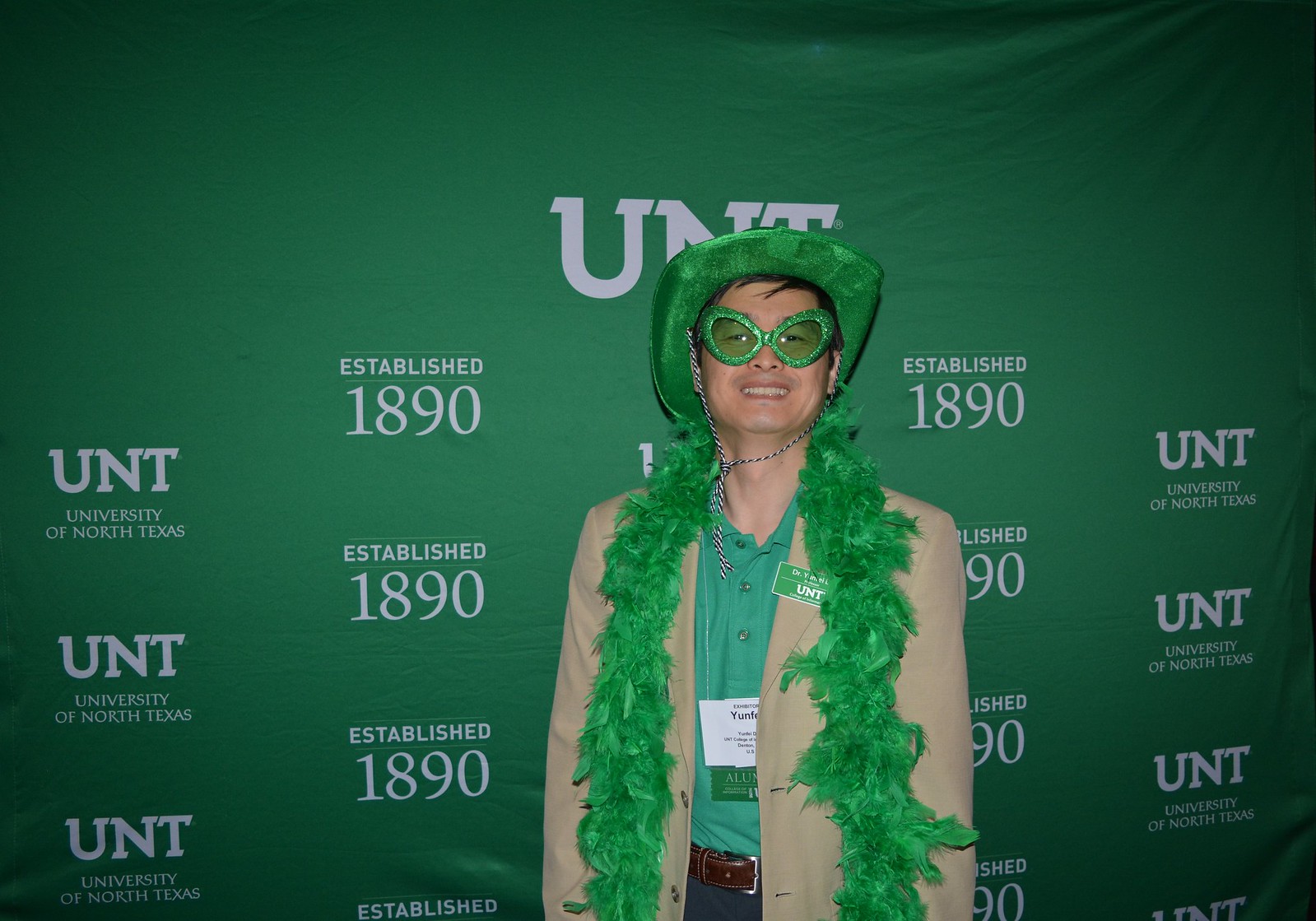The image features an Asian man wearing a vivid green polo shirt paired with dress pants that are partly obscured. A brown belt secures the dress pants. He sports a light beige overcoat, worn open to display the shirt, with a green name tag on the left side of the coat labeled "UNT" in white capital letters. Draped around his neck is a flamboyant green feather boa that cascades down his front, adding a playful flair to his attire. He wears a large smile and tops off his ensemble with a green velvet cowboy hat, complete with a black and white chinstrap. His look is completed with oversized, green, sparkly costume sunglasses. The backdrop behind him is entirely green and prominently features the white text "UNT" at the top. Further rows alternate between "UNT University of North Texas" and "Established 1890," repeating in a seamless pattern.